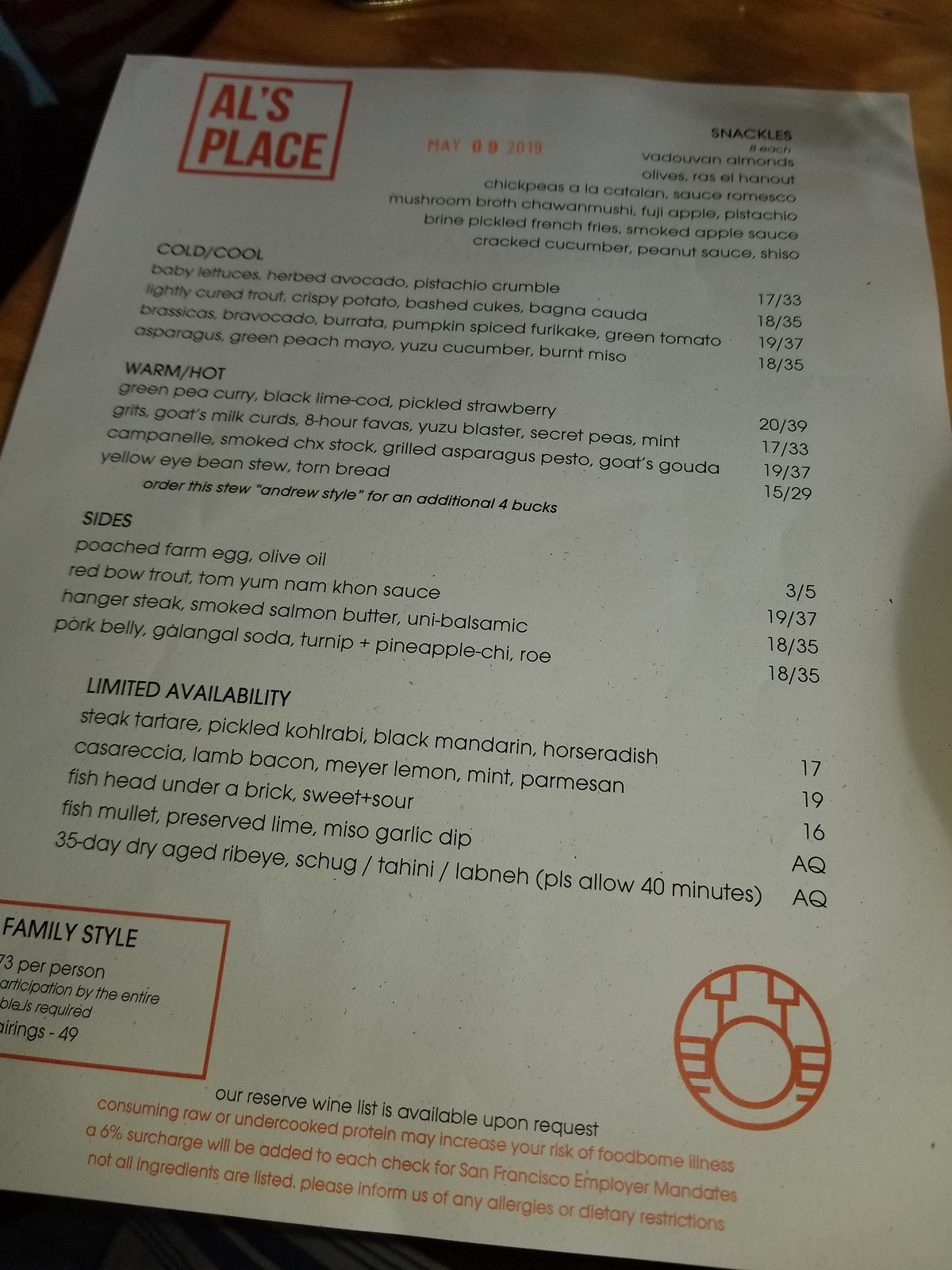A detailed menu from Owl's Place, dated May 9th, is prominently displayed. At the top, the menu is divided into sections: "Snackles," "Cold & Cool," "Warm/Hot," "Sides," and "Limited Availability." 

Under the "Cold & Cool" section, some featured items include:
- Baby lettuces with herbed avocados and pistachio crumble, priced at $17 or $33,
- Lightly cured trout paired with crispy potato, bashed cukes, and baña cauda, available for $18 or $35.

In the "Warm/Hot" section, notable offerings are:
- Green pea curry with black lime and cod, accompanied by pickled strawberry, costing $20 or $39.

Among the "Sides," there is a:
- Poached farm egg in olive oil, with prices set at $3 or $5.

On the bottom left of the menu, there's a partial view of a box detailing "Family Style" options along with the price per person.